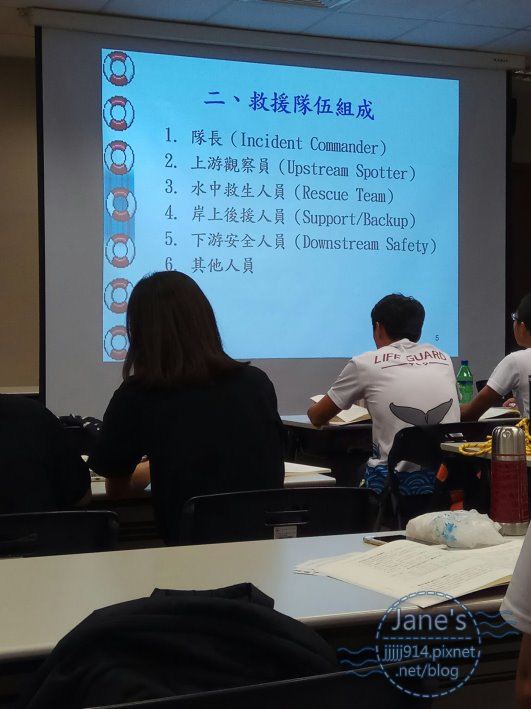The photograph captures a classroom or conference setting from the perspective of a seated participant. In the foreground, rows of two-seater desks populate the room, each with open books or pamphlets on them. A few individuals with dark hair are seated at these desks, all wearing casual clothing, and their attention is directed towards a large overhead projector screen at the front. The person standing at the head of the room has "Lifeguard" written on the back of their shirt, suggesting a training or safety briefing. The screen displays a bulleted list, numbered one through six, presented in both Chinese (or Japanese) and English. The list includes titles such as Incident Commander, Upstream Spotter, Rescue Team, Support/Backup, Downstream Safety, while the sixth item lacks an English translation. Additionally, life preservers are depicted along the left side of the presentation, emphasizing a water safety theme.